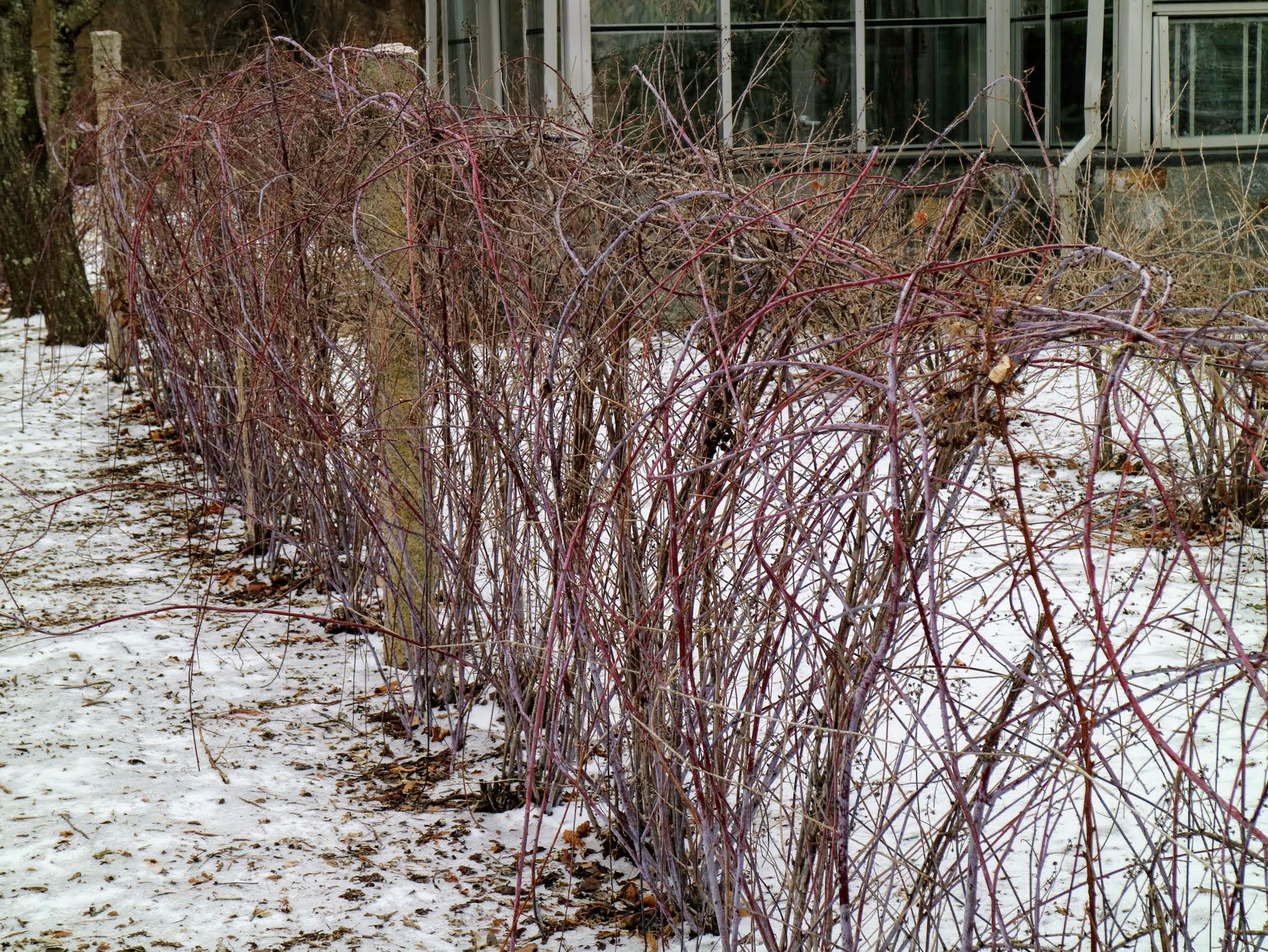The photo captures a snowy winter scene, dominated by a metal fence entwined with reddish-brown vines that almost obscure its structure. Three wooden posts sporadically emerge from the ground, supporting the vine-covered fence. The backdrop features a house or a residential building with an apparent sunroom or patio made largely of glass, visible only in part. The ground is coated with lightly dirty snow, with patches of exposed earth and scattered lawn debris further emphasizing the winter setting. In the distance, faint outlines of tree bark are discernible against the otherwise subdued landscape, enhancing the quiet, wintry atmosphere of the scene.